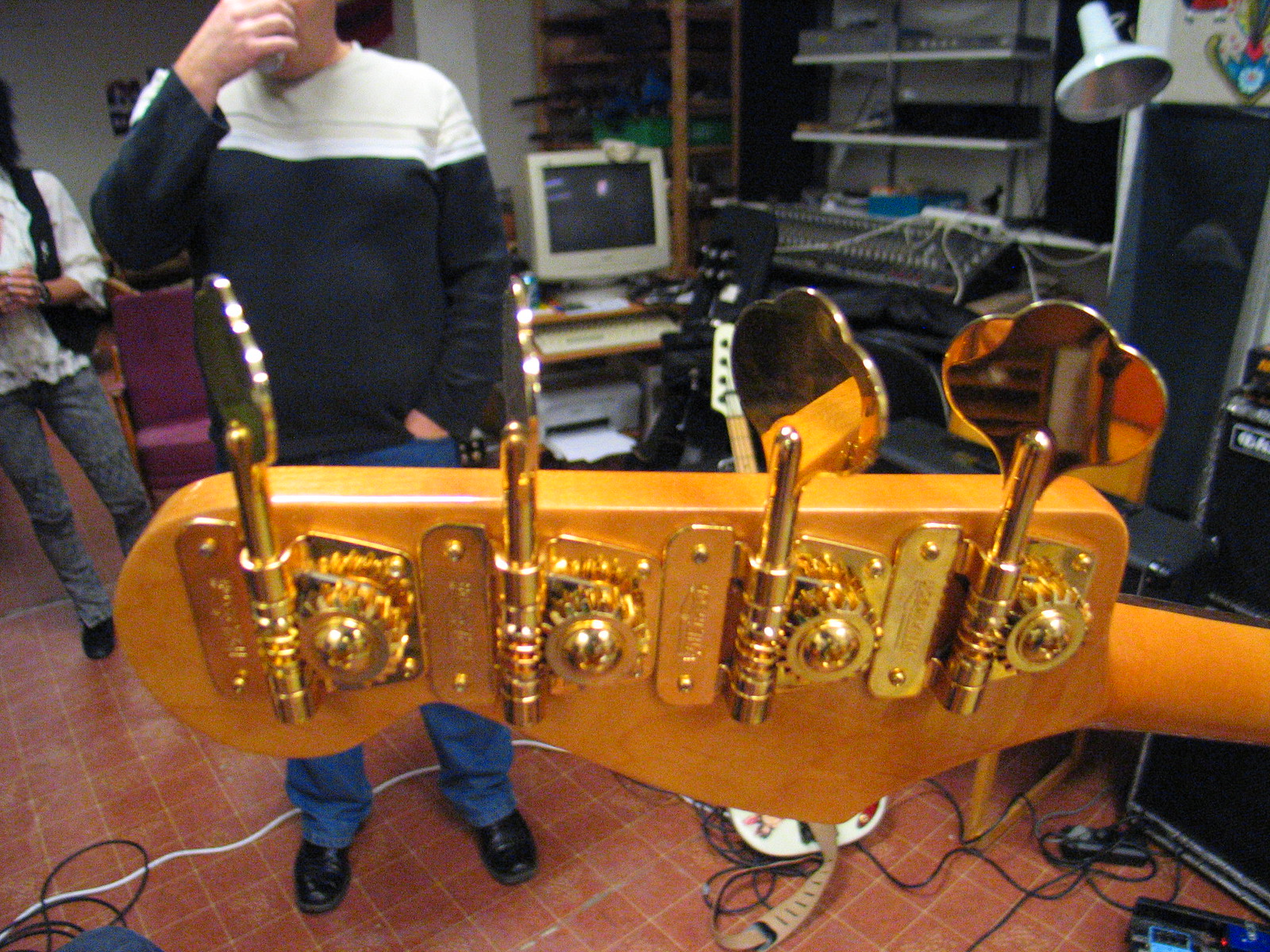The image centers on a close-up view of the headstock of a four-string bass guitar, highlighting the gold-colored tuning knobs, likely not made of real gold. The headstock and a portion of the neck, which appears to be crafted from a tan maple wood, dominate the forefront. This live image captures the intricate details of the guitar's machine heads and strings.

In the background, the setting unfolds as a music studio filled with various pieces of equipment. A computer monitor and keyboard are visible, as well as a shelf holding other musical gear, including what looks like a large amplifier. To the right, another guitar is partially visible, showing its string-playing area and a strap for support. Wires snake across the floor, connecting the equipment.

Additionally, there are two figures in the room. The first is a man with black shoes and jeans, drinking from a cup with his right hand, while his left hand rests in his pocket. Behind him, another person stands, whose gender is indeterminate due to the head being cut off from the image. The room is also furnished with a few chairs, emphasizing its purpose as a functional and busy recording or music-making space.